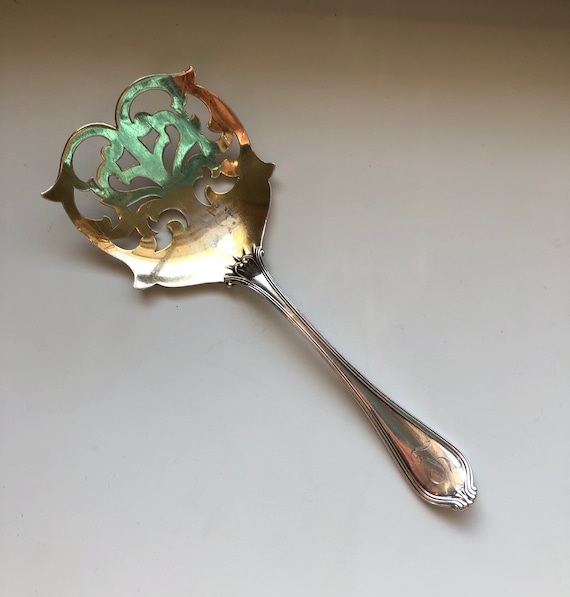This image depicts an intricate, antique cucumber server, primarily crafted from sterling silver with a glossy, silvery finish. The handle is smooth and tapers elegantly towards a heart-shaped serving end, featuring an elaborate vine-like pattern with carved-out sections that add to its distinctive appearance. The tip of the server exhibits a greenish hue, with hints of yellow oxidation suggesting its ancient origins. The top side of the server displays curves and holes that, while aesthetically pleasing, render it impractical for holding liquids. The utensil is set against a light gray background, with slight copper undertones visible at the top, further enhancing the rich detailing of this elegant and historical piece. The server appears to be part of a larger, unseen set, accentuating its antique and ornate design.